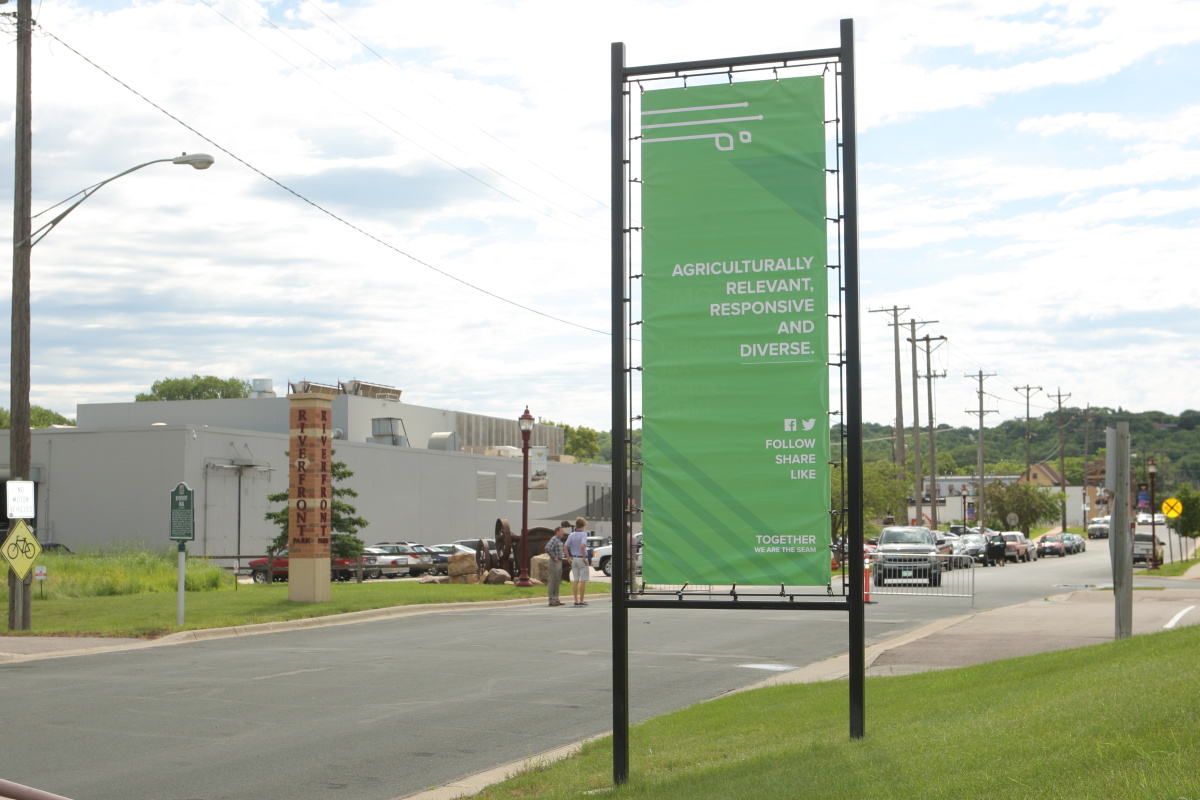A vibrant image portrays a clear day with a bright turquoise-blue sky dotted with white clouds. The focal point is a green sign set within a sturdy black frame, akin to a stake planted firmly in the grassy embankment along a road. The sign prominently displays the words "Agriculturally Relevant," "Responsive," and "Diverse," along with social media commands: "Follow, Share, Like." At the bottom, the text reads, "Together We Are The Seam," though some words are less legible due to the small font size. The top of the sign features three horizontal lines embellished with tiny leaf designs. Surrounding the scene, there are various details illustrating a dynamic environment: parked and traveling cars on the road, a distant gray building with a brown post in front, numerous power lines crisscrossing above, a yellow railroad crossing sign, and a bicycle crossing sign. The setting further includes a lavish display of green grass and trees, juxtaposed with a dense forest backdrop and a light pole extending electrical wires down the road. Additionally, there are two individuals standing on the street, observing the approaching car, and a distinct brick signpost on the far side inscribed with "Riverfront Park."